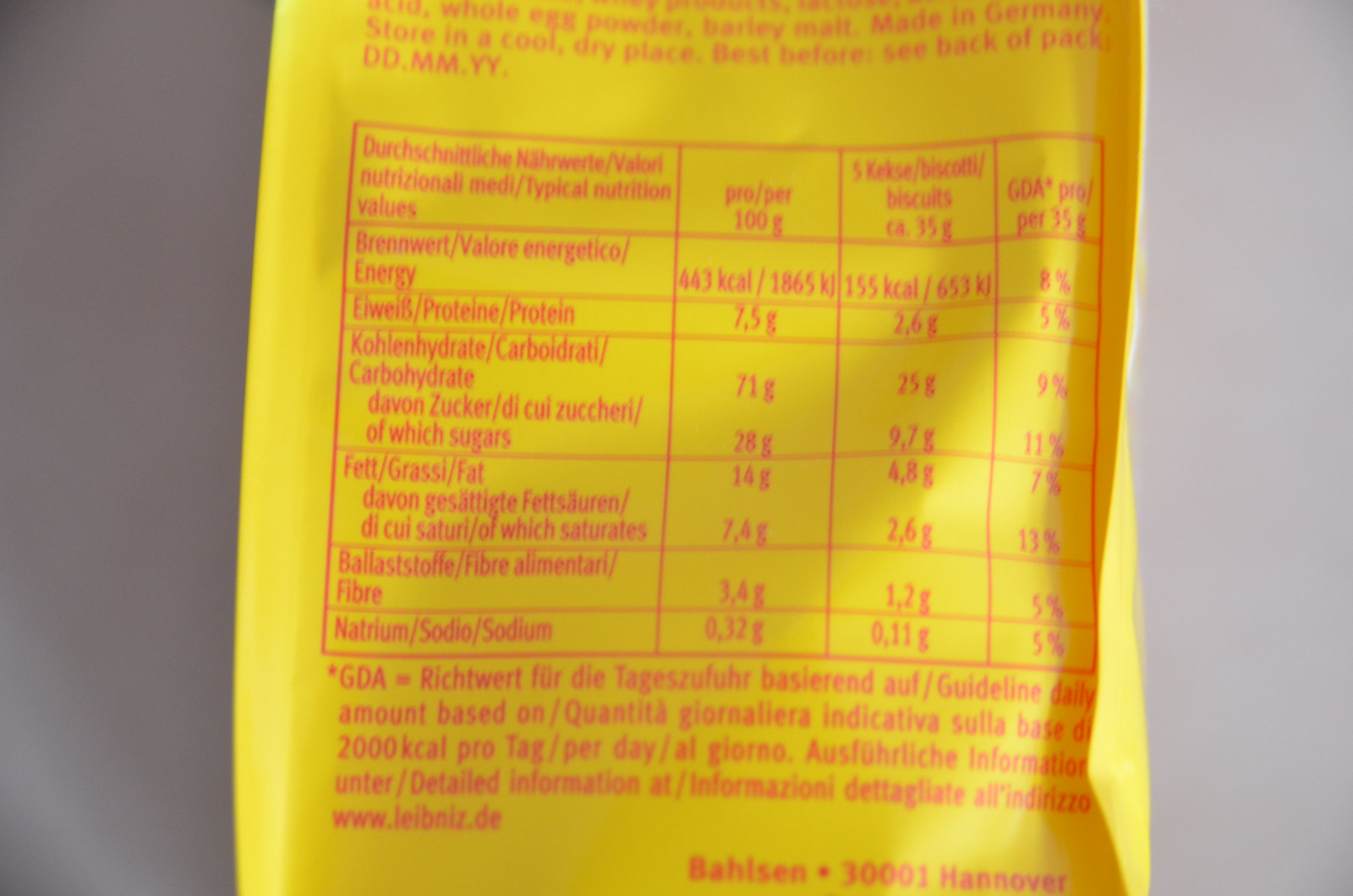This close-up image focuses on the backside of a yellow food package, taking up 75% of the frame. The photograph is zoomed in to highlight the detailed nutritional information on the package. At the top, there is a paragraph written in pinkish-colored text. Below this, four categories are organized in a square-framed outline.

Each category features names on the left side; the English word is listed with its translation in another language directly above it. To the right, values are provided per 100 grams, followed by values for five biscuits, and then the GDA per 35, each label precisely marked. Beneath this section, there is a phrase starting with "GDA equals," followed by a series of non-English text in pink. Further down, the package reads "BAHLSEN 30001, Hanover." The image has a light gray background on both the left and right sides, adding contrast to the package.